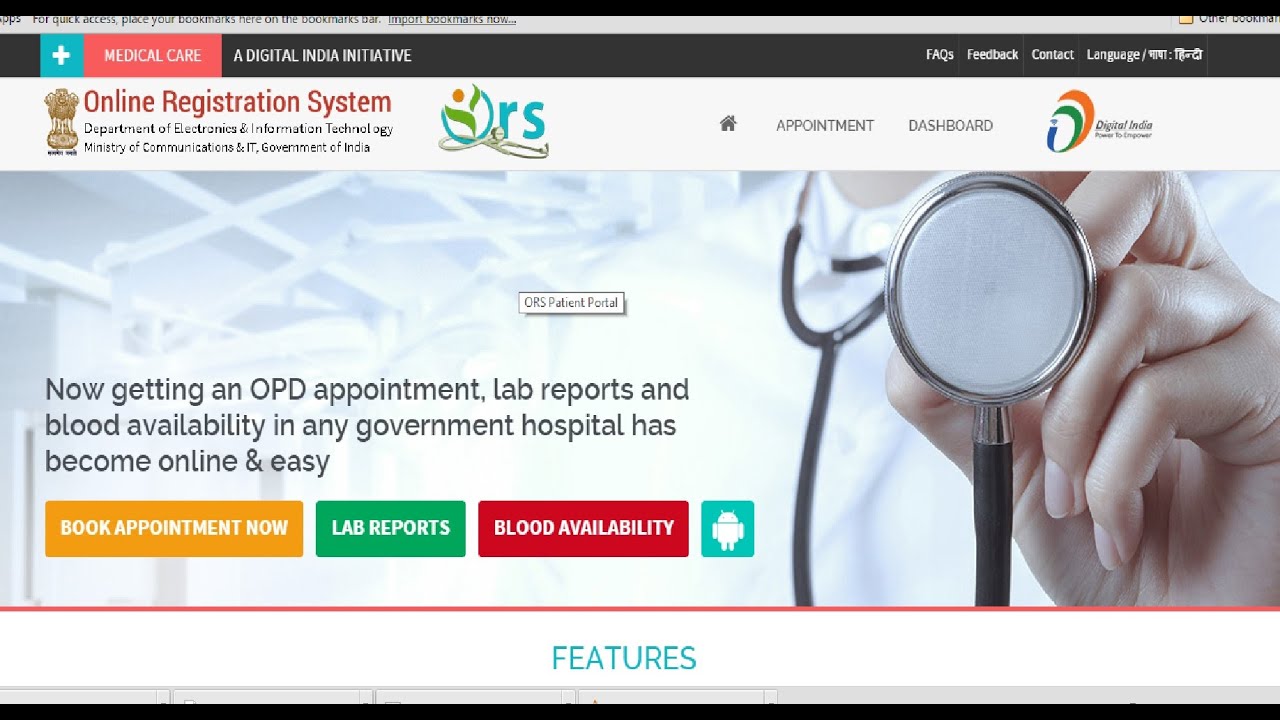This is a detailed descriptive caption for the image:

The screen capture displays a computer monitor against a stark white background, prominently showing an online registration system interface. At the top left corner, there is a blue square icon with a white cross, adjacent to a red rectangle labeled "Medical Care." To the right of this red rectangle, a black bar extends across the screen's right side, bearing the text "Digital India Initiative" in white. 

On the upper right, typical menu options are visible, including "Fax," "Help," and more. Directly below these menu buttons, the text "Online Registration System" appears in red. Beneath this, the full title reads: "Department of Electronics and Information Technology, Ministry of Communications and IT, Government of India."

The central portion of the screen captures a wide image stretching from left to right. On the right side of this image, there is a close-up view of a physician's neck and chest area, noticeably highlighted by the stethoscope draped around their neck. The physician holds the stethoscope's bell in their left hand, turned towards the viewer.

On the left side of this central image, text announces, "Now getting an OPD appointment, lab reports, and blood availability in any government hospital has become online and easy." Below this statement, three distinct buttons are displayed: an orange button labeled "Book Appointment Now," a green button labeled "Lab Reports," and a red button labeled "Blood Availability."

At the bottom, separated by a horizontal red line extending across the screen, is the heading "Features" written in blue text.